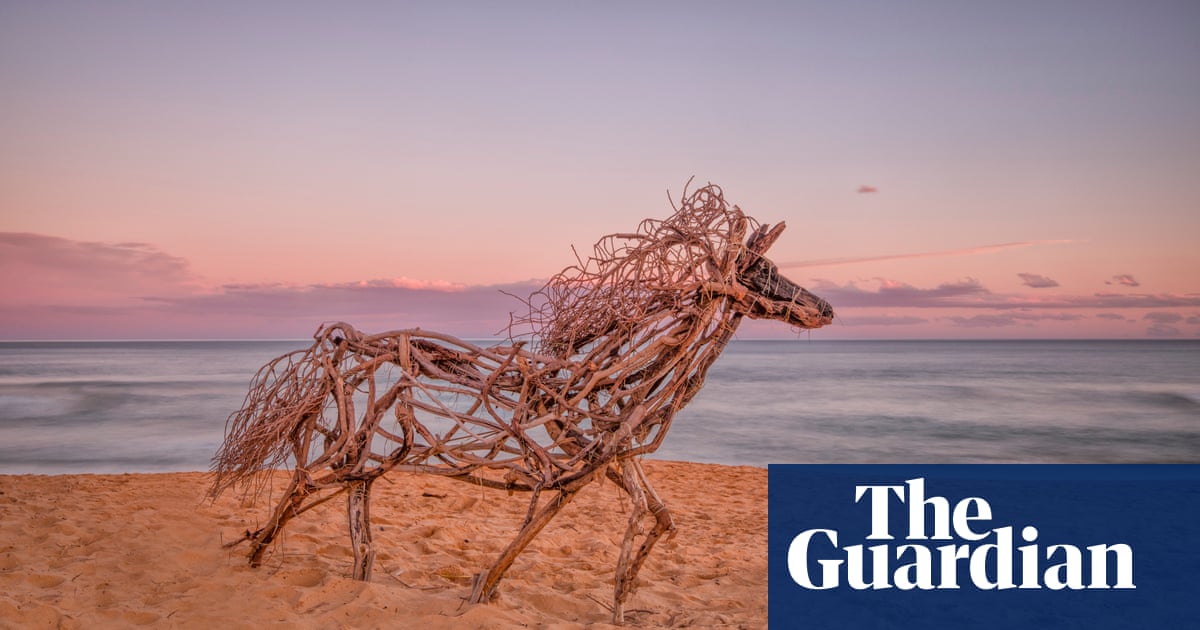The image is a detailed, color photograph of a beach at sunset, published on The Guardian's website, marked by a prominent blue rectangle with white text reading "The Guardian" in the bottom right corner. The beach has a sandy, beigey-brown terrain, disrupted by numerous footprints, giving it a textured look. In the foreground stands a remarkable art installation of a horse, crafted meticulously from driftwood, sticks, twigs, and straw-like materials. This sculpture, which appears to be running, features a darker brown head and a wild mane made from vines and branches. The legs of the horse are embedded in the sand, providing stability, and the tail resembles an upside-down branch, adding an intricate touch to the natural composition. The background captures a serene ocean with bluish-gray waves under a softly glowing pastel sunset sky, blending hues of light blue, pink, and orange, with clouds adding depth to the horizon.